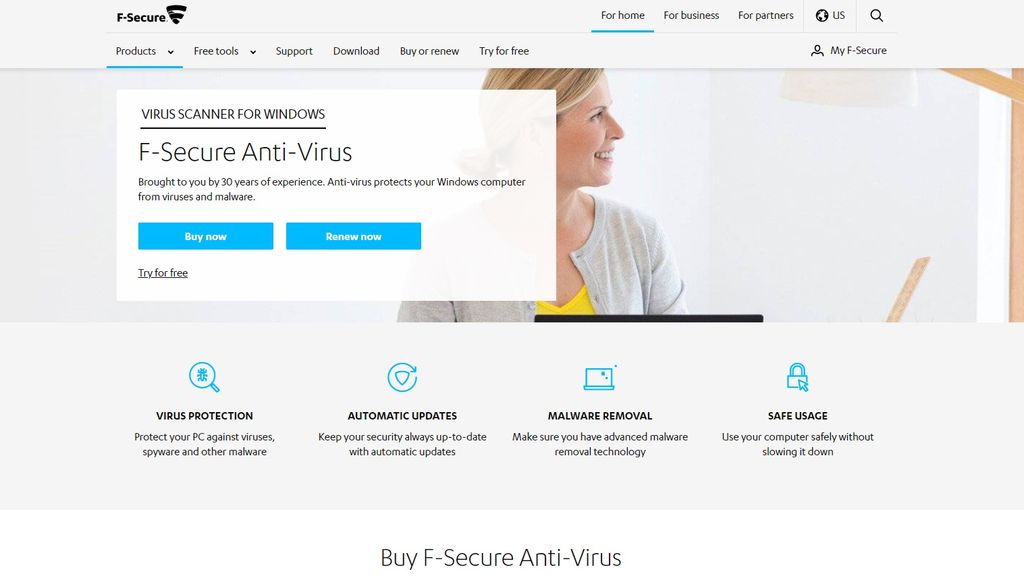In this image, we have a screenshot set against a white background. At the upper left corner, bold block text displays "F-Secure." Toward the upper right, there are navigation options listed: "For Home," "For Business," "For Partners," along with "U.S." adjacent to an illustrated planet Earth icon. Below these options, the menu includes "Products," "Free Tools," "Support," "Download," "Buy or Renew," and "Try for Free."

The central part of the image features a photo of a woman appearing to be in her 30s. She has blonde hair pulled back and is wearing a sweater. Her gaze is directed to the east (right side of the screen). Partially covering the back of her head is a text box that reads: "Virus Scanner for Windows, F-Secure Anti-Virus."

Further down the image, a detailed description states: "Brought to you by 30 years of experience, F-Secure Anti-Virus protects your Windows computer from viruses and malware." Following this, options are presented to either "Buy Now," "Renew Now," or "Try for Free."

At the very bottom of the screen, bold text directs: "Buy F-Secure Anti-Virus."